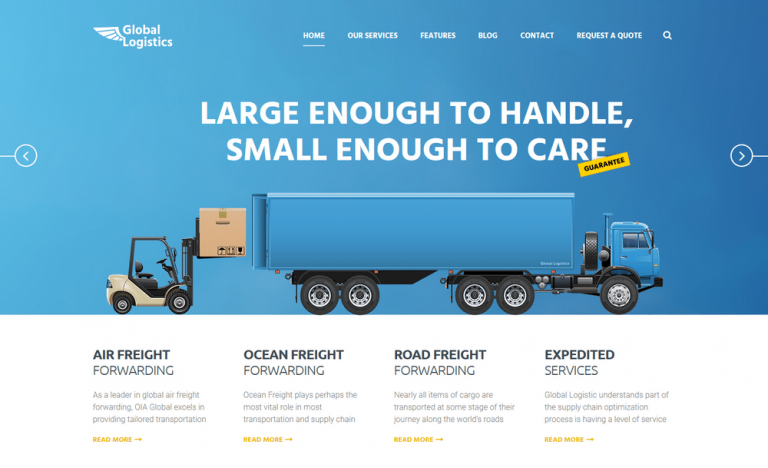This screenshot captures the homepage of a logistics company's website. At the top, the words "Global Logistics" are prominently displayed, with a stylized white wing emerging from the word "Logistics". Below this heading, a vast blue background mimicking the sky dominates most of the screen.

In the foreground, there is a striking image of a large blue container truck. The truck is equipped with a blue cab and has five wheels, including an additional tire behind the cab. Positioned at the rear of the truck is a box lift, underscoring the vehicle’s capability to handle substantial cargo.

Written prominently on the image is the company's slogan: "Large enough to handle, small enough to care. Guaranteed."

At the top of the page, there is a navigation menu featuring the following options: Home, Our Services, Features, Blog, Contact, Request a Quote, along with a search bar.

Toward the bottom of the screen, the website offers detailed service options including:

- **Air Freight Forwarding**: "As a leader in global air freight forwarding, OIA Global excels in providing tailored transportation." There is a "Read more" button for additional information.
- **Ocean Freight Forwarding**: "Plays perhaps the most vital role in most transportation supply chain." Again, a "Read more" button is available for further details.
- **Road Freight Forwarding**
- **Expedited Services**

Each service option includes a brief description and a "Read more" link for users to explore further details.